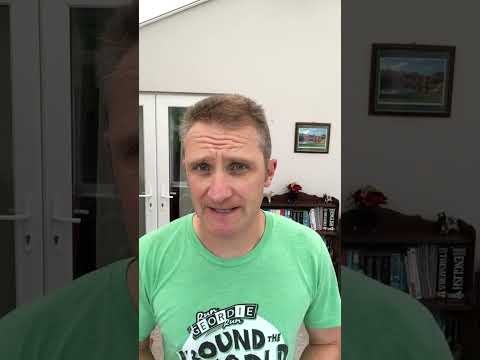The image depicts a middle-aged white man, likely in his 30s or early 40s, with short light brown hair and a concerned expression. He is seen mid-word with his eyebrows knitted together, and his mouth partially open. He is wearing a light green short-sleeved t-shirt that features the word "GEORDIE" in large letters at the top and "Around the World" inside a large white circle below, with a silhouette of a person in the "O" of "World." The man has no facial hair and is gesturing with his hands in front of him, his left wrist adorned with a black wristwatch. The background reveals he is indoors, with large glass French doors behind his left shoulder and a light beige wall featuring a framed picture. To the right, there is a small bookcase filled with books. The photo has a thick black border on both sides.